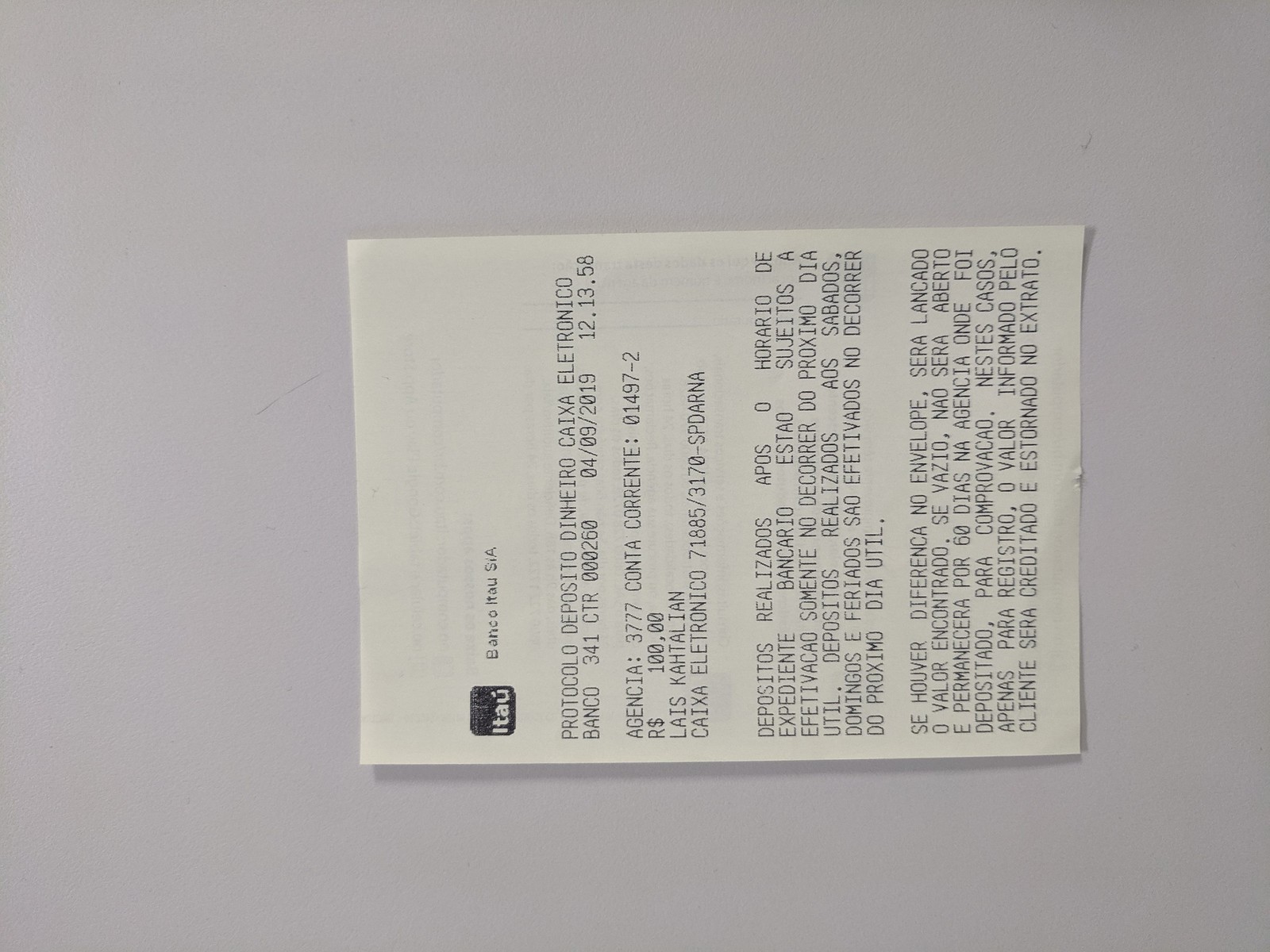In the image, we observe a gray table or countertop. Prominently placed across it is a white piece of paper, resembling a receipt from a bank. The paper is oriented horizontally, with the top facing the left side of the image and the bottom towards the right. At the top of the receipt, the words "Banco Itao S.A." are clearly visible. Accompanying the text is an icon or logo with the word "Itao" enclosed within a black square, positioned in the upper left corner. The text appears to be in a foreign language, and reads, in part, "Protocolo Deposito Dinero Caixa Electronico." The date on the receipt is "12-04-09-2019," and it indicates a transaction amount of "$100,00."